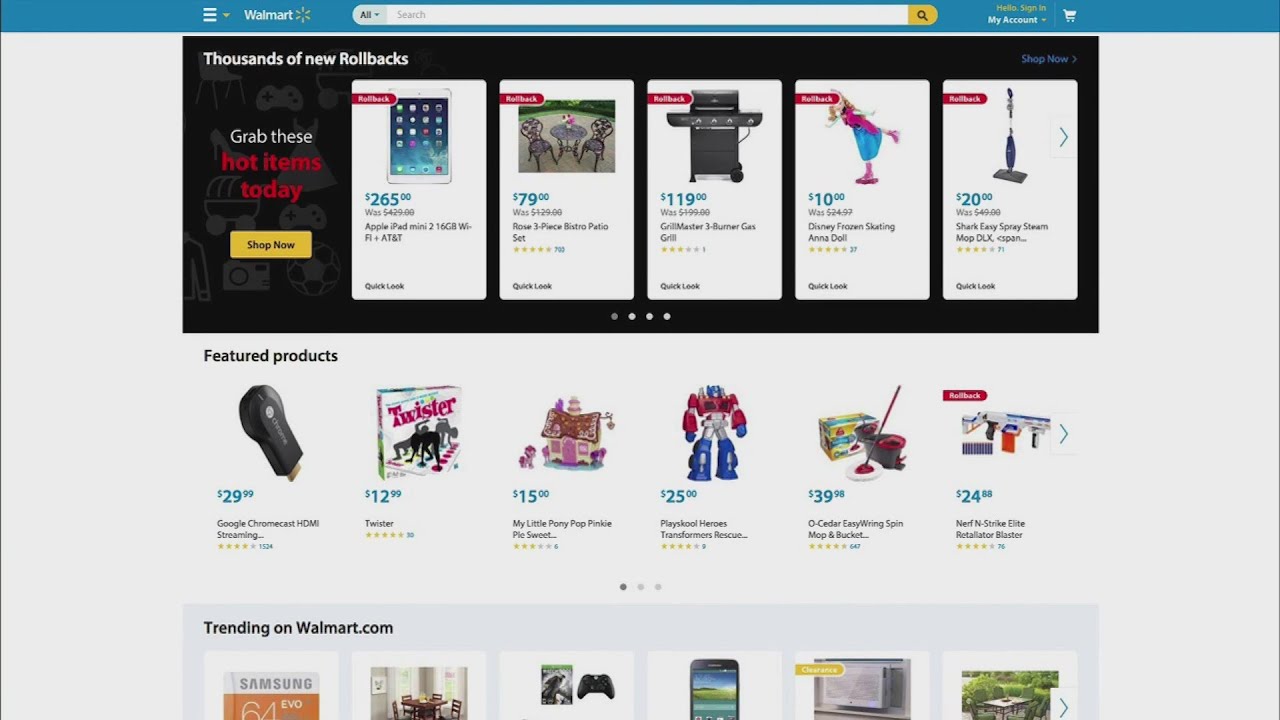This is a detailed caption describing a sales webpage for Walmart products:

"At the top of the Walmart sales page, a prominent menu announces, 'Thousands of new rollbacks. Grab these hot items today.' Highlighted in this section are five prime products: an Apple iPad, a bistro set, an outdoor gas grill, a Disney doll from the movie Frozen, and a Shark Easy Spray steam mop. These are the key promotions featured prominently. Below this, another row titled 'Featured Products' showcases six items: a Google Chromecast HDMI streaming dongle priced at $29.99, a Twister game for $12.99, a My Little Pony Pop Pinkie Pie suite priced at $15 (name partially cut off), a PlaySchool Heroes Transformer Rescue toy priced at $25 (name partially cut off), an Oseeter Easy Ring Spin Mop and Bucket for $39.98, and a Nerf N-Strike Elite Retaliator Blaster at $24.88. Beneath this, there's a row with trending items on Walmart. However, the icons are cut off midway, making it impossible to discern the names or prices of these products, only the tops of the icons are visible."